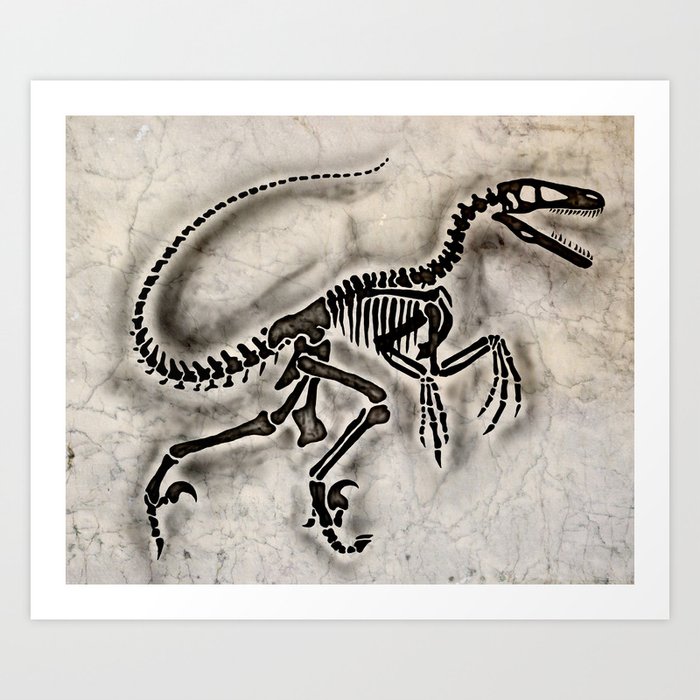The image depicts an artistic black-and-white drawing of a dinosaur skeleton, likely a raptor such as a Velociraptor, displayed in a vertically rectangular format with thick gray borders on the top and bottom, and a distinct white border inside that. The background resembles whitish marble with intricate gray veins and scattered black dots, giving it an elegant yet eerie appearance. The dinosaur's skeletal structure is detailed, featuring long arms with three elongated fingers ending in sharp, nail-like claws. It stands upright, supported by its back legs, with its front limbs poised in the air. The tail is notably long and curves back towards the middle of its head, adding a sense of dynamic movement to the composition. The skull is characterized by a prominent eye socket and menacing blackened teeth, as if marked with ink. The overall depiction suggests the dinosaur is still animate, captured mid-motion in a striking profile view.